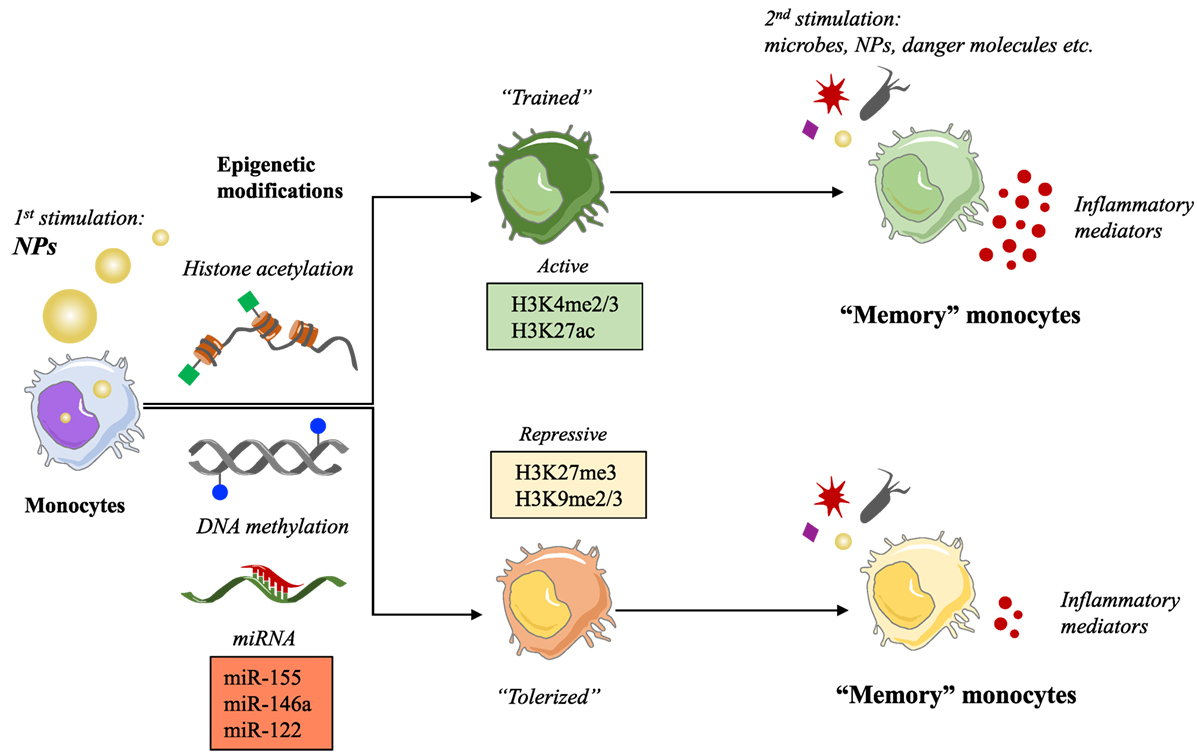The diagram depicts a cellular process with detailed stages and epigenetic modifications, set against a white background without a border. On the left side, it starts with the first simulation, where "NPs" (in bold capital letters) are represented by three gold circles. Below this, an irregularly shaped round object labeled "monocytes" connects with lines branching into two sections to the right.

The top section is labeled "trained" and features a green irregularly shaped object. This section includes detailed descriptions like H3K4ME2, H3K27AC, and references to histone acetylation. This trained cell then undergoes a second stimulation involving "microbes, NPs, danger molecules, etc.," and transforms into memory monocytes, shown as a green cell with many tiny red circles surrounding it. Above this are further descriptions such as "inflammatory mediators."

The bottom section, labeled "tolerized," shows a coral-colored object with a yellow center and mentions repressive markers like H3K27ME3, H3K9ME2, and the term "polarized." This cell also responds to stimulation, proceeding to become a memory monocyte depicted as a yellow cell with numerous red dots around it. Similar to the top section, the term "inflammatory mediators" is present here as well.

Additional textual elements include black text annotations, various epigenetic markers, and modifications illustrated through squiggly lines, brown yo-yos, green squares, gray DNA with blue dots, and some silvery black and red lines, contributing to the detailed process of cellular changes.